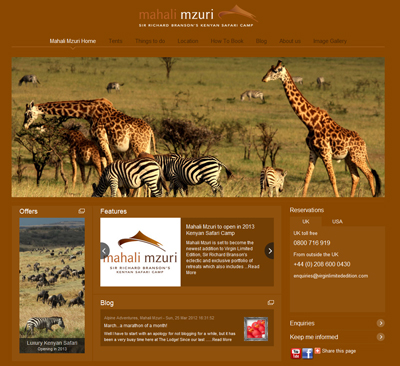The image is a square with a reddish-brown background. At the top, there is a heading that reads "Mahali, Missouri" in a lighter shade of reddish-brown. Right below it, "MZURI" is written in white font. There is a line of small print following the text, but it is difficult to discern. An icon is present nearby, though its details are unclear.

Beneath the heading, the words "Mahali, Missouri home" are prominently displayed in white. Additional readable text includes "Things to do," "Blog," "Image gallery," and possibly "About." 

Across the center of the image, a rectangular section features a scenic view of the Serengeti with visible wildlife. Two large giraffes and two black-and-white zebras stand out, with another zebra in the background that has a brownish tint. Other, indistinct animals can be seen further in the background as well.

In the bottom left corner, there are some offers showcasing more animals and a clickable blog square. Additional information appears on the right side of the image, including the option to stay informed with "Keep me informed" and the ability to select between the UK or USA.

There's also a row of social media icons for YouTube, Facebook, and one unrecognized platform, accompanied by a "Share this page" prompt.